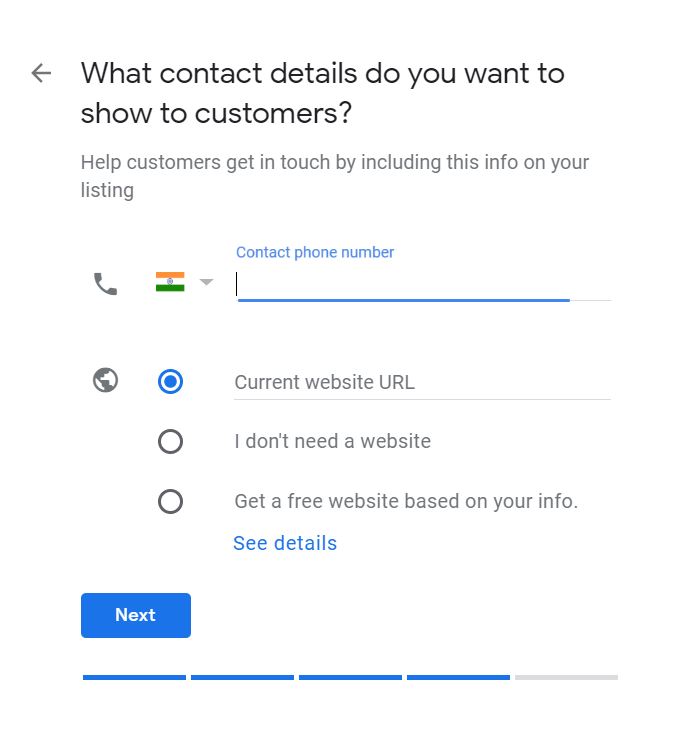The image appears to be a screenshot from a mobile phone or a webpage interface, designed to help users provide contact details for their business listings. 

At the top, there is a navigation arrow pointing left, possibly indicating a way to return to the previous page. The main heading reads "What contact details do you want to show customers?" followed by a question mark. Directly under this heading, a subtext in gray states, "Help customers get in touch by including this info on your listing."

Below this subtext, the visual components of the contact details form are arranged sequentially:
1. A telephone symbol is shown next to a drop-down menu that allows users to select their country by flag.
2. To the right of this, in blue text, is the label "Contact phone number," accompanied by a field where users can input their phone number.
3. Further down, there's a globe icon next to the label "Current website URL," with a pre-selected radio button indicating that this option is currently active.
4. Below this, there are two additional options with radio buttons that are not selected: "I don't need a website" and "Get a free website based on your info. See details."

At the bottom of the form, there is a "Next" button. Beneath this button, a progress indicator bar consists of five segments, where the first four segments are filled in blue and the last segment remains gray.

The entire form is set against a white background, suggesting a clean and simple layout designed to guide users through the process of updating their contact information. The overall purpose of this interface is to allow users to specify how they would like to be contacted by customers, providing various options to ensure comprehensive and accurate contact details.